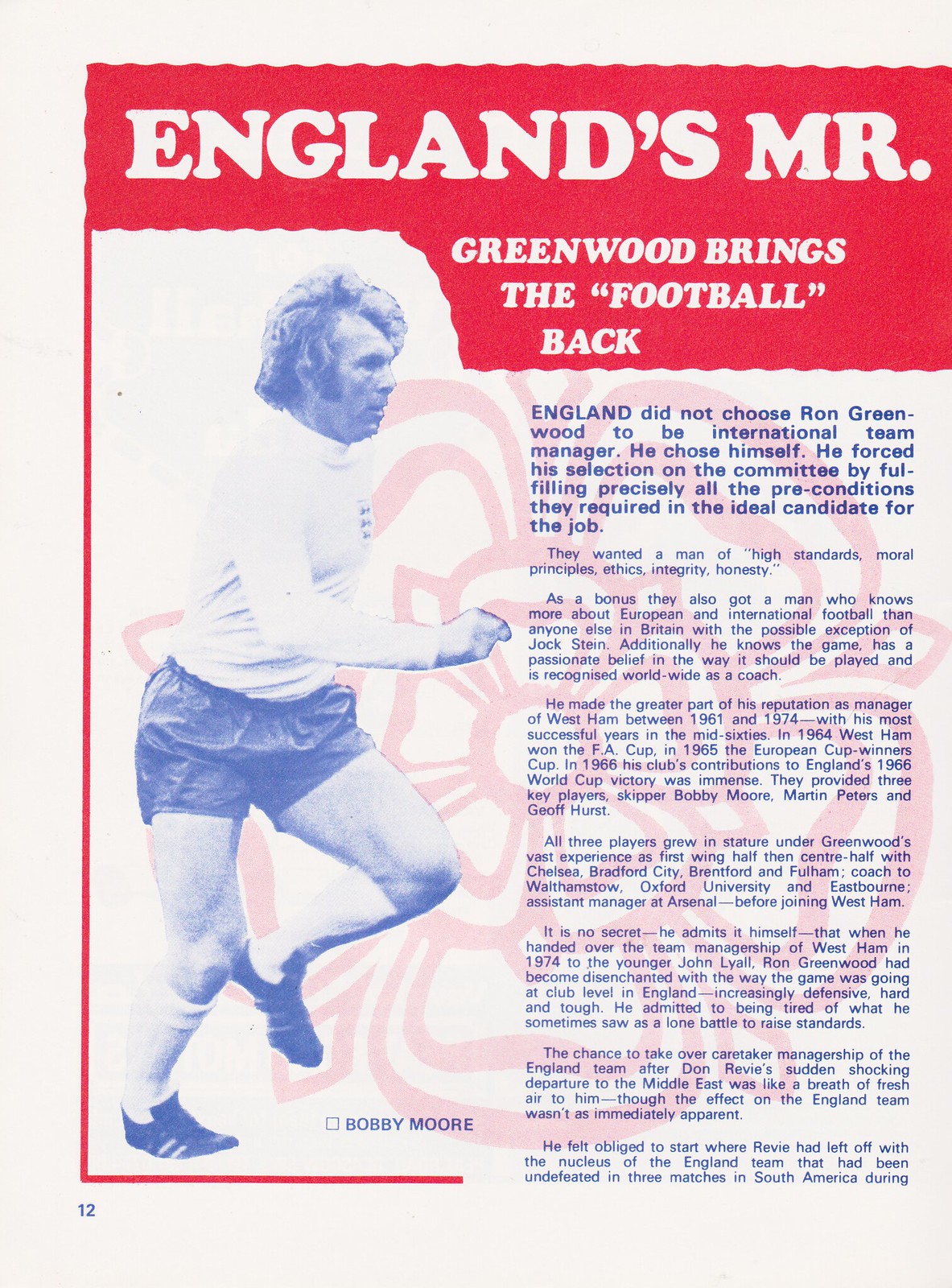This image is a vintage page from a sports magazine or program, bordered in red with a blue-ink illustration and text. Heading within a red highlighted box reads, "England's Mr. Greenwood brings the football back." On the left side is a picture of Bobby Moore, identified by the caption, wearing a white long-sleeved jersey, dark shorts, white socks, and black football shoes. A pink floral watermark overlays the image. The article details how Ron Greenwood became the England international team manager by meeting all the committee's ideals, emphasizing his high standards, moral principles, ethics, integrity, and honesty. Greenwood, who built his reputation leading West Ham from 1961 to 1974, taking them to several victories including the FA Cup (1964) and European Cup Winners’ Cup (1965), replaced Don Revie under sudden circumstances. Disenchanted by the defensive play at club level, Greenwood saw the caretaker role as a fresh start, continuing where Revie left off with an undefeated team from South America. Page number 12 is displayed in the lower-left corner.